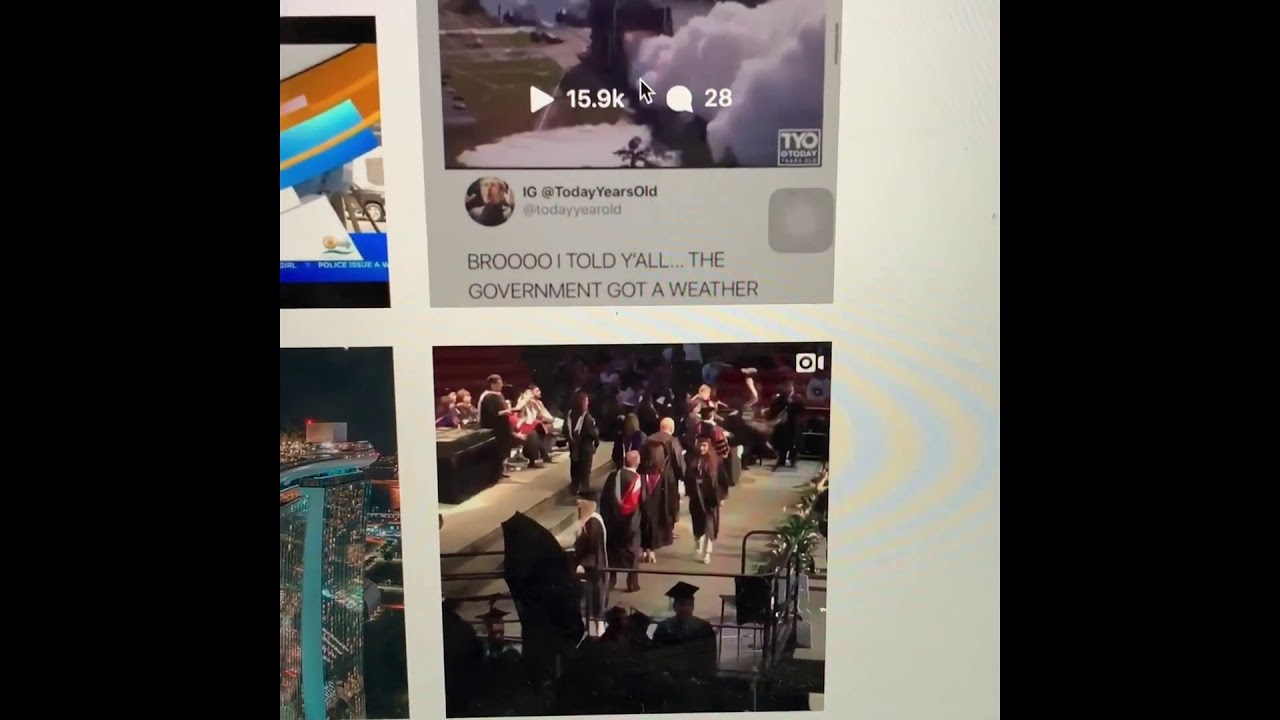The image appears to be a screenshot of an Instagram feed displayed within a rectangular frame, longer on the horizontal axis. On either side of the frame, there are black strips. In the middle of the frame are two rows of images; the images on the left side are partially cut off, while those on the right side are fully visible. Both rows are separated and bordered by white space.

At the top of the visible feed, there is a post indicating "15.9k plays" and "28 comments." This post seems to include text that reads "IG, today years old, at years old, bro, I told y'all the government got a weather," and what appears to be a photo of snow, though the image is partially cut off. The second post, beneath the first, shows a group of people in caps and gowns, likely at a graduation ceremony, walking on a stage. The crowd and the lower parts of the image are not visible. An Instagram logo is positioned in the upper-right corner of the display, suggesting this is a screenshot of an Instagram page. The overall context suggests the viewer is not very familiar with Instagram.